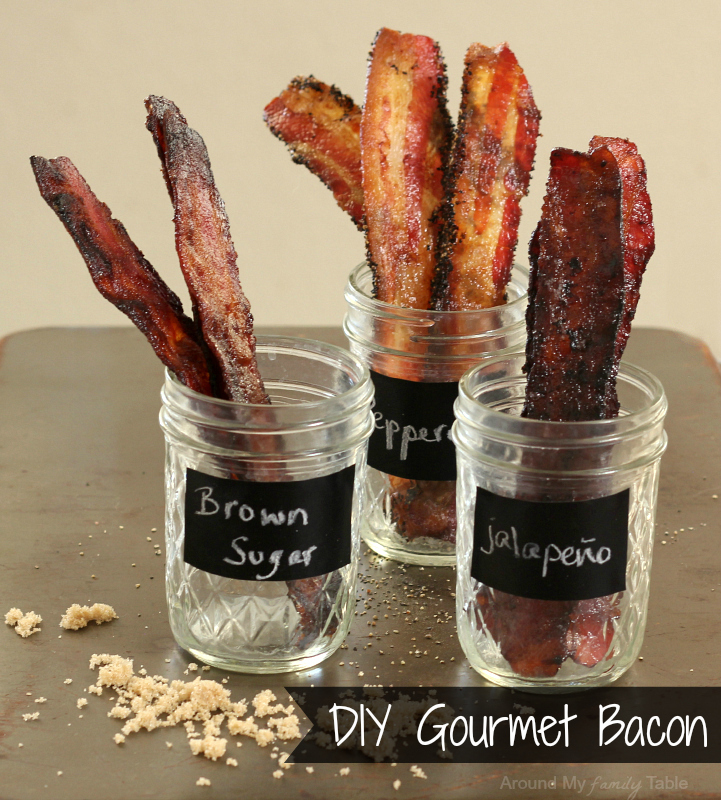In this portrait-oriented image, three transparent pint-sized Ball jars are neatly arranged on a dark brown table, each jar prominently featuring a black label with white handwritten text. The label on the front-left jar reads "brown sugar" and contains crispy, upright bacon strips with a darkened edge, resembling beef jerky. Behind it, another jar marked "pepperoni" holds lighter, reddish bacon, also vertically oriented. To the right, the third jar's black label displays "jalapeno," showcasing more reddish-brown bacon strips.

Scattered in front of the jars are crumbs of brown sugar and pepper, adding texture to the scene. In the bottom right corner, the words "DIY gourmet bacon" appear in a white handwritten font on a semi-transparent black banner. Below this, a gray watermark reads "around my family table," with "family" slanted in italics. The light gray background wall contrasts with the detailed focus on the table and its contents, highlighting the artisanal presentation of this gourmet bacon assortment.